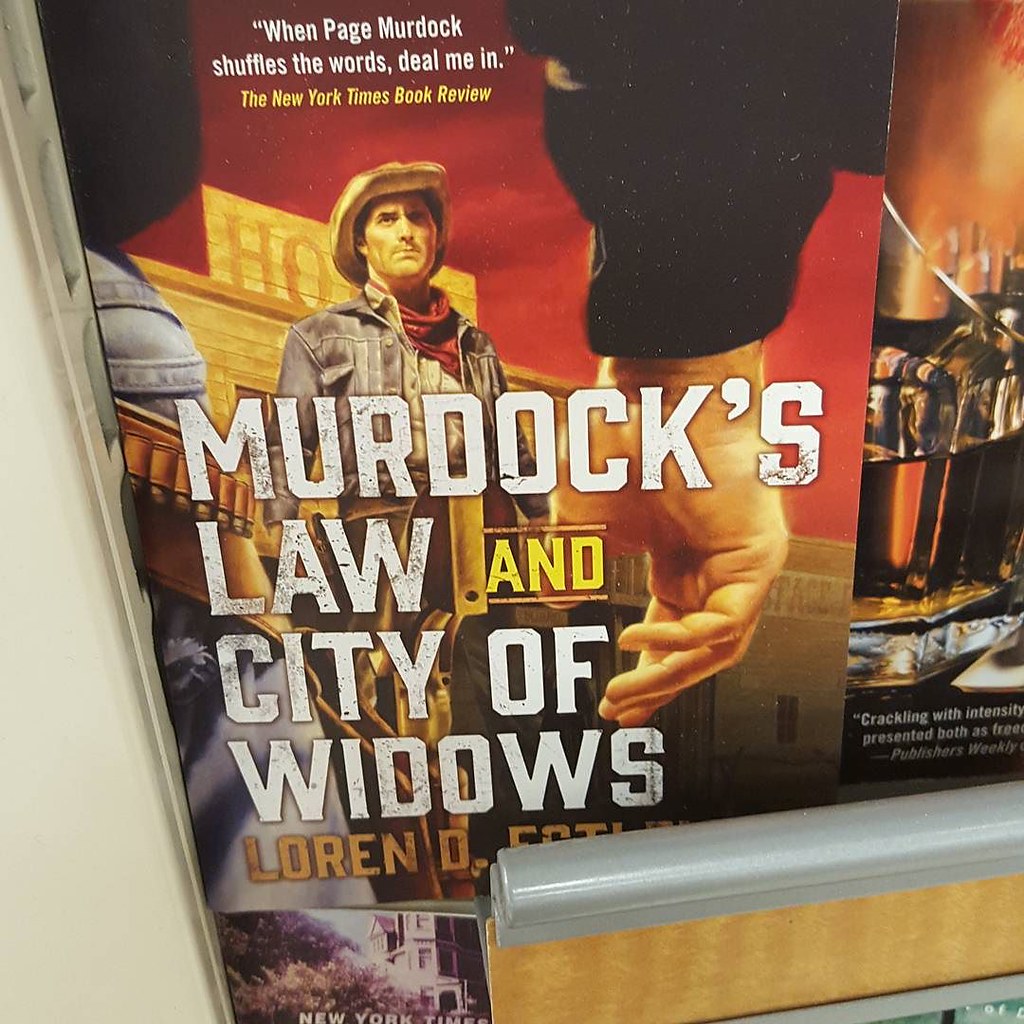In the image, the main focus is a book prominently positioned in the center. The cover features a vivid, full-color illustration depicting a scene from the Old West. The background of the book's cover shows a fiery red sky behind an old-style building with a partially obscured sign that reads "hotel." A rugged cowboy stands in front, wearing a jean jacket, white shirt, red handkerchief, and a worn hat. To the left of the cowboy, a close-up of someone's pants with a gun belt is visible, with their arm extending to the right side, clad in a dark long-sleeve shirt. The title on the cover reads "Murdoch's Law and City of Widows" in white and yellow text, attributed to Lauren D., though some of the text is obscured by a shelf.

The setting appears to be indoors, likely within a bookstore. Along the left side of the image, there is a beige structure resembling a shelf or wall, and at the bottom right, a silver and wooden barrier secures the book in place on the shelf. The colors in the scene include white, off-white, yellow, red, orange, black, purple, gray, brown, and tan, creating a rich and engaging visual palette. The overall scene suggests a detailed and immersive book display, inviting viewers to explore the narrative of an Old West adventure.